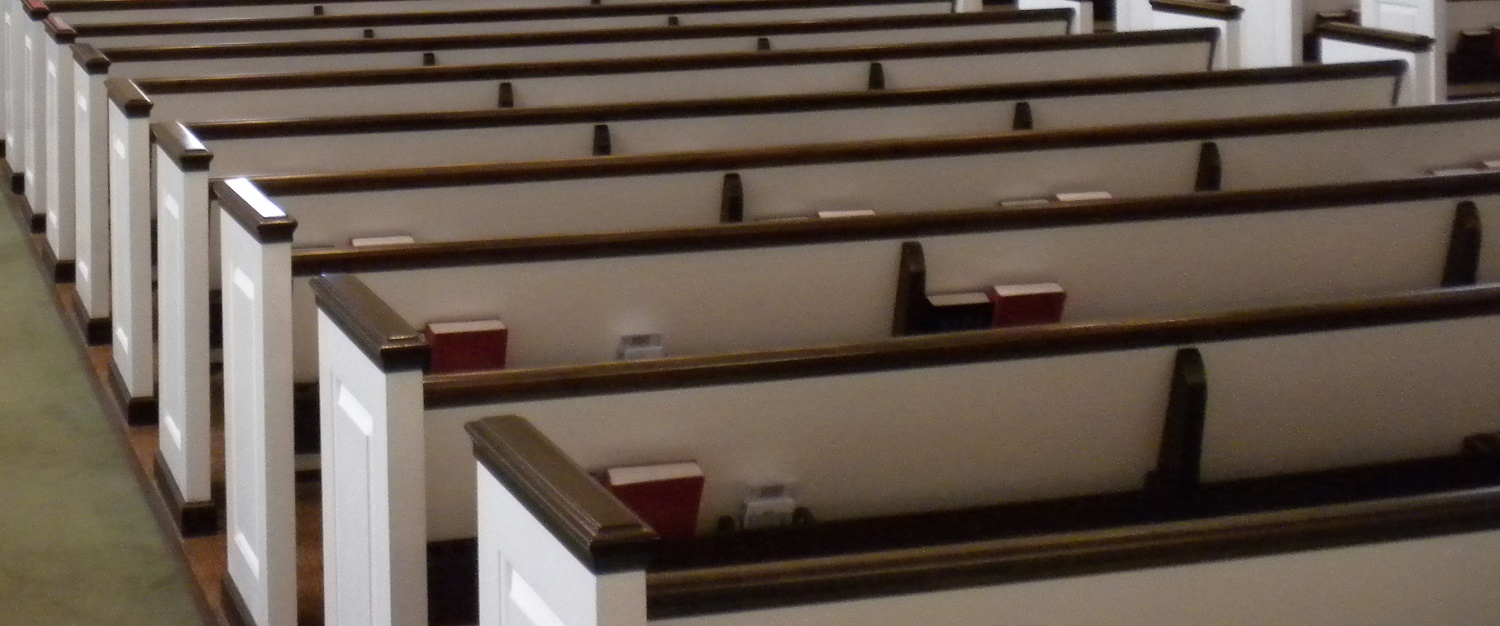The image features a horizontal photograph of a church interior, showcasing a row of predominantly white wooden pews. The pews are meticulously aligned, extending toward the upper left corner of the image, and totaling around nine or ten visible pews. Each pew is characterized by a stark white color with contrasting dark brown elements, including straight-edged armrests and a top ridge along the backrest. The floor beneath the pews is coated in an orangish-brown hue, while a gray-green carpet runs parallel to the pews on the left side of the image. Nestled in the backrests of the pews are several hymnals; some are red with white pages, and others appear darker, possibly black or brown.